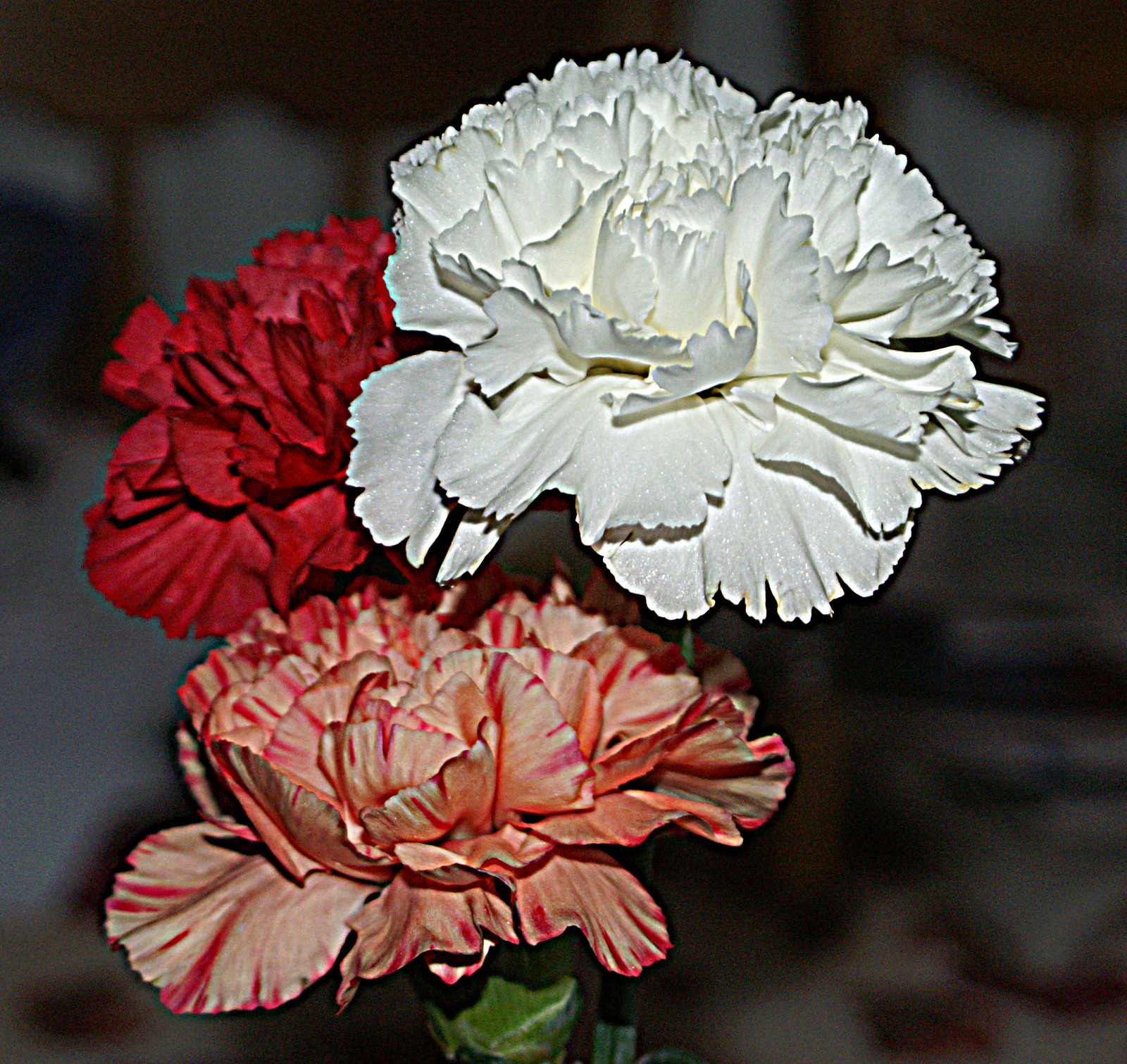The image features a close-up of three vibrant carnation flowers, dominating more than half of the frame against a blurred, indistinct background with splotches of white, brown, and hints of wood. The upper right blossom is a large, bright white carnation with intricate, scalloped petals that show shadows and indentations. To its left, partially obscured, is a dark burgundy red carnation, adding a deep, rich hue to the composition. Below these, a pink carnation with variegated patterns of white and pink streaks displays a unique, almost striped appearance. Visible green stems extend from the flowers, hinting at leaves, which add a touch of natural greenery to the scene.